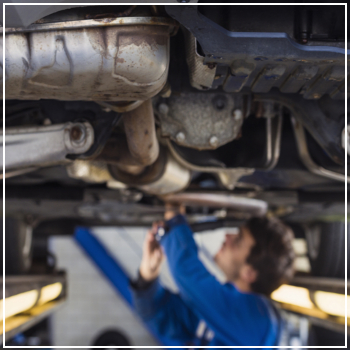In this detailed square-shaped photograph, a mechanic with short, curly brown hair and light skin, dressed in a blue jumpsuit, is depicted working underneath a vehicle in an indoor auto shop. The image, framed by a thin white border, reveals the mechanic looking upwards with both hands immersed in the vehicle's undercarriage. The area around the mechanic is well-lit by large yellow lights positioned on either side, likely attached to a small lift visible in the shot, which also contains tires. Although the specific vehicle type is unclear, various gray metal parts and bits of tubing can be seen around the mechanic's hands, suggesting he might be fixing the oil filter. The bottom portion of the square photo appears blurred, while the top portion captures the detailed metalwork of the vehicle's underside.